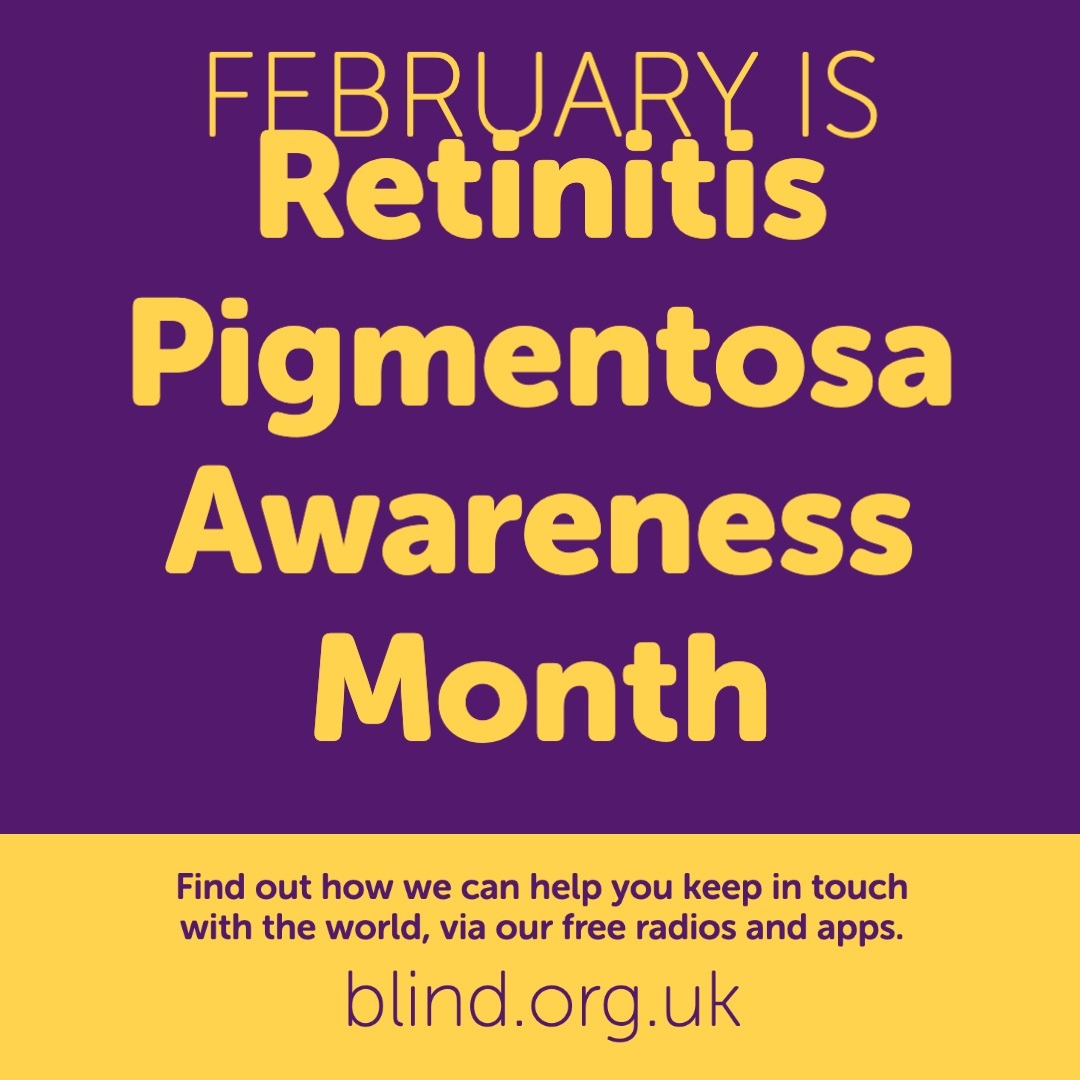This is an image of a public service announcement from Blink.org.uk for Retinitis Pigmentosa Awareness Month. The advertisement features a bold, square design with a prominent purple background and a bright yellow stripe at the bottom. The upper portion displays yellow text that reads "February is Retinitis Pigmentosa Awareness Month" in eye-catching, large bubble letters, while the lower yellow stripe contains purple text that invites viewers to "Find out how we can help you keep in touch with the world via our free radios and apps." The URL "Blink.org.uk" is featured in purple below this message. The advertisement is purely graphical, without any photographic elements, people, animals, buildings, or vehicles. This clean, text-based design ensures that the message is clear and attention-grabbing.